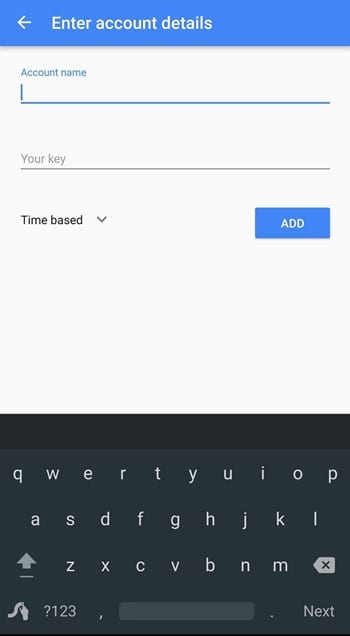**Detailed Caption:**

This image is a screenshot of a simplistic login screen, likely captured from a smartphone, either an Android or an iPhone. At the very top, there is a header bar in a distinctive shade of blue, reminiscent of Microsoft's default color palette. The heading text within the bar is pure white, reading "Enter Account Details," accompanied by a left-pointing white arrow, suggesting navigation or a return to a previous screen.

Directly below the header, in prominent blue font, the text "Account Name" is visible, marked by a blinking cursor, indicating that the field is active and ready for input. Adjacent to this text field is a solid line where users can type in their account name. Beneath this, there is a light gray horizontal line which separates the sections.

Next, there is a prompt in muted gray text, "Your Key," which implies that users should enter their password or security key in this field. Beneath this key input area, there is a dropdown menu with the selection "Time-based" displayed, suggesting the capability to choose alternative configurations through additional options that would appear upon interaction. To the right of this dropdown, there is a prominent blue button labeled "ADD" in all capital, white letters, designed to add or confirm the inputted information.

At the bottom of the screen, a standard virtual keyboard is visible in black, ready for users to type in their credentials. The user interface is designed to guide the user through an orderly login process with clear and intuitive prompts.